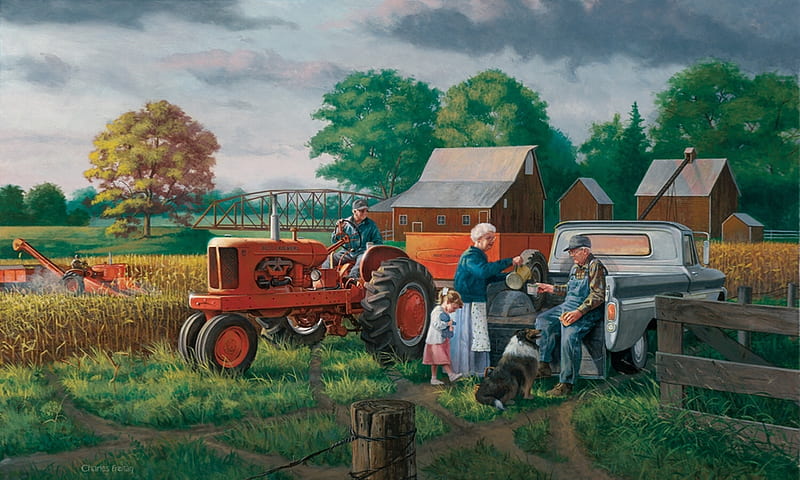This is a highly detailed and realistic color painting of a serene farm scene, capturing the essence of rural life. At the center, an older man wearing overalls and a wide-brimmed hat sits on the bed of his pickup truck, which is parked in the middle of a golden wheat field. An elderly woman with white hair, dressed in a green coat, a light blue skirt, and a white polka-dotted apron, is pouring water from a pitcher into his cup. Beside her stands a little girl in a pink dress holding a doll, her hair neatly styled in pigtails adorned with scrunchies. 

In front of the truck, a large collie dog, resembling Lassie, sits attentively, looking up at the man. To the left, a man in a green jacket and sunglasses rides a red tractor with large black wheels, watching the scene unfold. Background elements include a red barn with a sloped roof, various pieces of farm equipment, a wooden fence, and a distant bridge surrounded by lush trees. The overall composition presents a picturesque, tranquil depiction of everyday farm life, capturing a moment of simple, heartfelt interaction amidst the pastoral beauty.